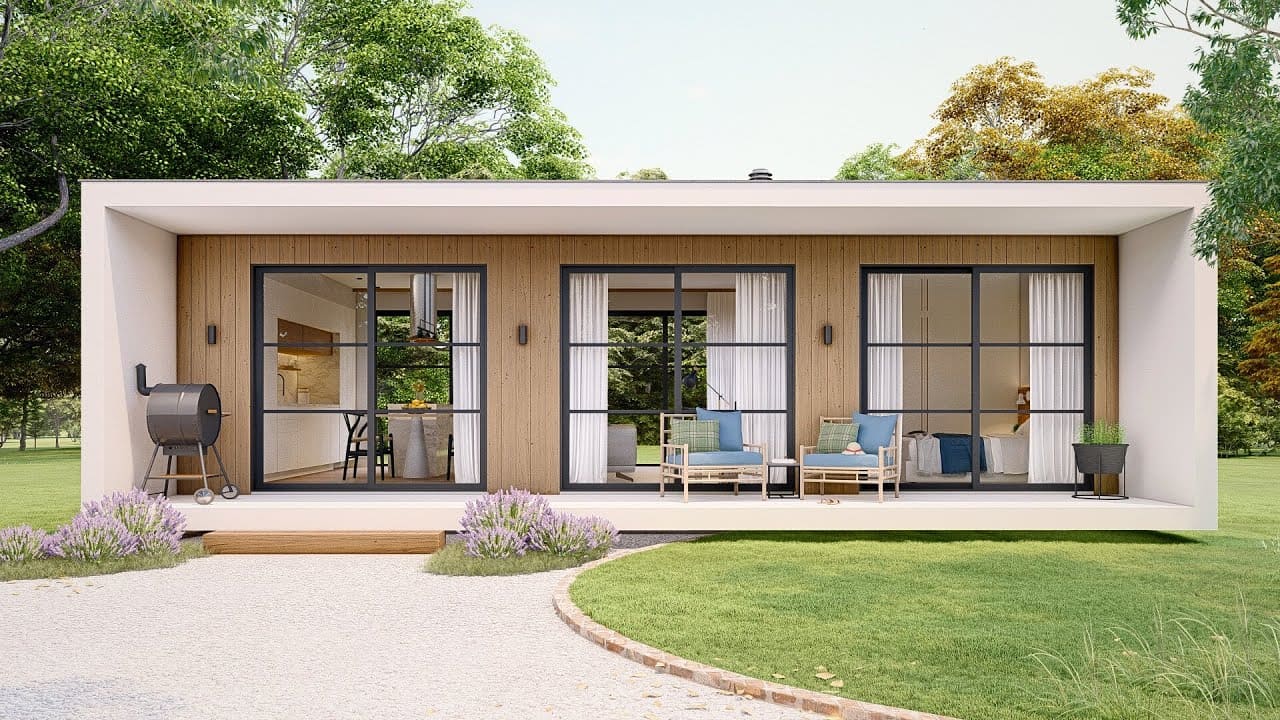In this image of a modern modular home, the rectangular structure stands prominently with its white, wood-look paneled finish, accented by light brown trims around three large, black-framed windows at the front. The windows are organized in a grid pattern, revealing glimpses of a sleek white kitchen, a gray couch, and a bed inside. Outside, the patio is a sizable rectangle made of what appears to be white plaster, and it showcases a cozy setup with two beige armchairs, each featuring blue and green cushions. On the left side of the patio, a black charcoal grill, resembling a barrel drum on wheels, rests against the wall. In front of the patio, lavender bushes add a splash of color, complementing the immaculate green grass that edges a brick-lined driveway. The scene is set against a backdrop of tall, leafy trees and a clear, blue sky, suggesting a serene and picturesque environment.